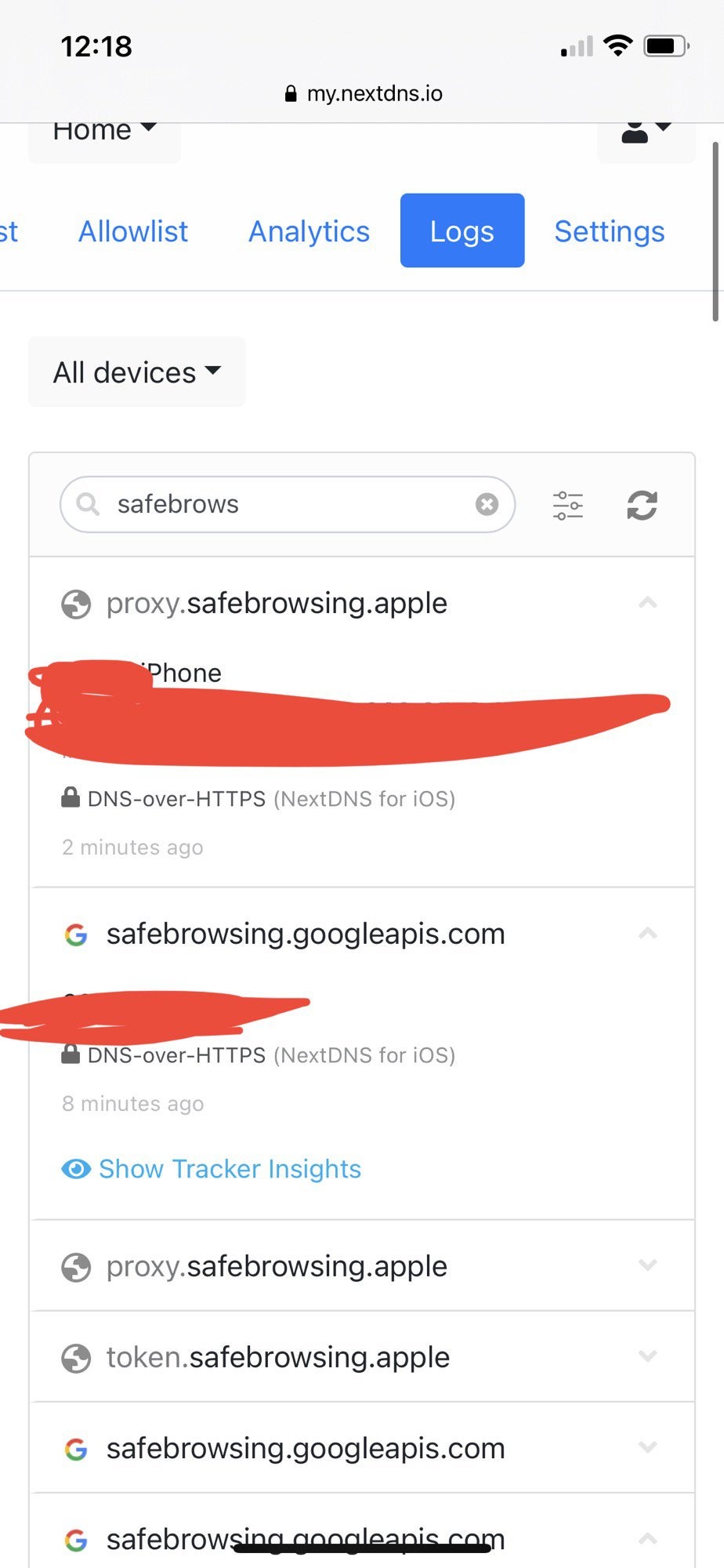Screenshot of a smartphone displaying the MyNextDNS.io interface:

At the top of the screen, the current time is shown as 12:18 in black text on the left, while the icons for Wi-Fi, cellular signal, and battery are positioned on the right. Below this status bar, the website URL "my.nextdns.io" is displayed prominently in the center, accompanied by a small lock icon on its left, indicating a secure connection.

The interface is segmented into several sections. Directly below the URL, navigation options are available, with a "Home" icon on the left and an "Account" icon on the right. The main menu is listed in blue font with the following options: Allow List, Analytics, Logs, and Settings. The "Logs" option is currently selected, as indicated by the blue box surrounding it.

Beneath the menu, a dropdown labeled "All Devices" appears, paired with a down arrow for device selection. Adjacent to this is a search field marked "Safe browse," flanked by a filter button and a refresh button.

The main content area features detailed logs:

1. The first entry shows "proxy.safebrowsing.apple" with a portion redacted by a red marker that likely obscures a phone number. The log notes "DNS over HTTPS" and timestamps the entry as "2 minutes ago."
2. The second entry lists "safebrowsing.googleapis.com" with another red marker obscuring part of the information, presumably a phone number, and also notes "DNS over HTTPS."

At the bottom of the log section, options in blue font prompt the user to "Show Tracker Insights," followed by a new set of entries:

1. "proxy.safebrowsing.apple"
2. "token.safebrowsing.apple"
3. "safebrowsing.googleapis.com"
4. "safebrowsing" with the rest of the domain obscured by a black line.

This comprehensive view of the MyNextDNS.io interface details the logs and filtering options available to users for managing their safe browsing settings.